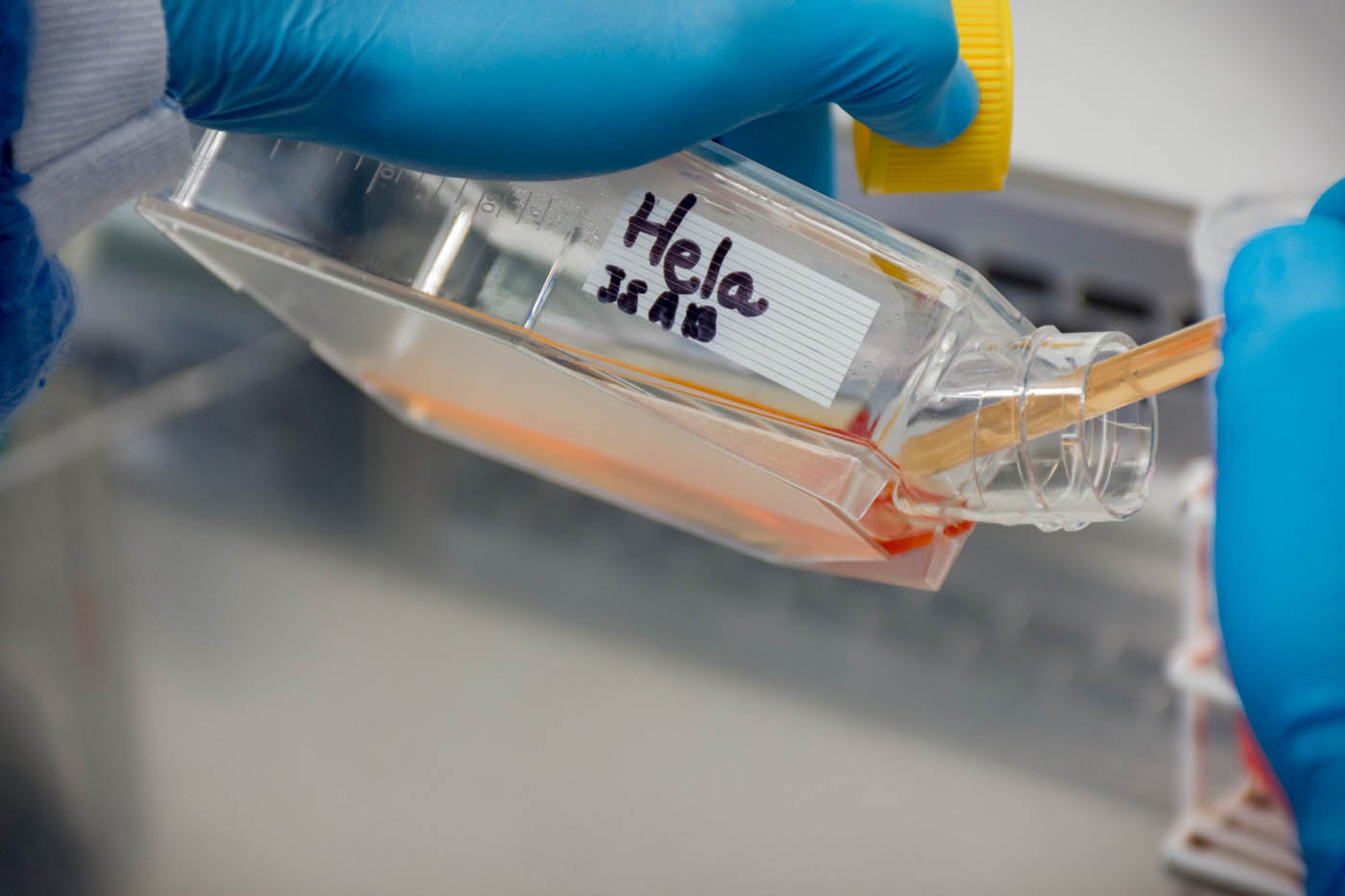A close-up image depicts a lab technician meticulously working in a laboratory setting. The technician is clad in a comprehensive decontamination suit, which includes blue latex gloves and a protective hood. The left wrist, partially visible, confirms the extent of the protective gear. They are handling a plastic container labeled "HeLa," with additional markings that are difficult to discern due to some blurriness. Using a pipette, the technician carefully extracts a sample from the container while holding its yellow cap in their left hand. The action seems to take place over a presumably stainless steel sink, although the exact details are blurry. In the background, a wire mesh container sheathed in blue rubber tubing is visible, likely intended for the storage or further analysis of the sample. The environment and equipment suggest a sterile setting, emphasizing the meticulous nature of the work being performed.